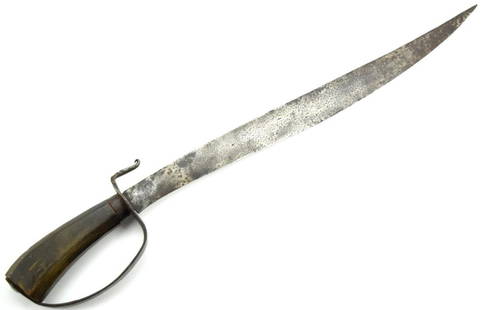The image depicts a weathered swashbuckler's sword, reminiscent of those used by pirates. Positioned horizontally against a white background, the sword extends diagonally across the scene. The handle, made of dark wood, is located on the left and features a circular metal guard that offers a secure grip for the hand. This guard, which curves up and to the left, allows for a thumb placement that enhances grip during a thrust. The slightly curved blade is long, narrow, and comes to a very sharp point. The blade appears tarnished and worn, displaying a mottled silver shade with patches of gray, black, and white, hinting at its age and extensive use.